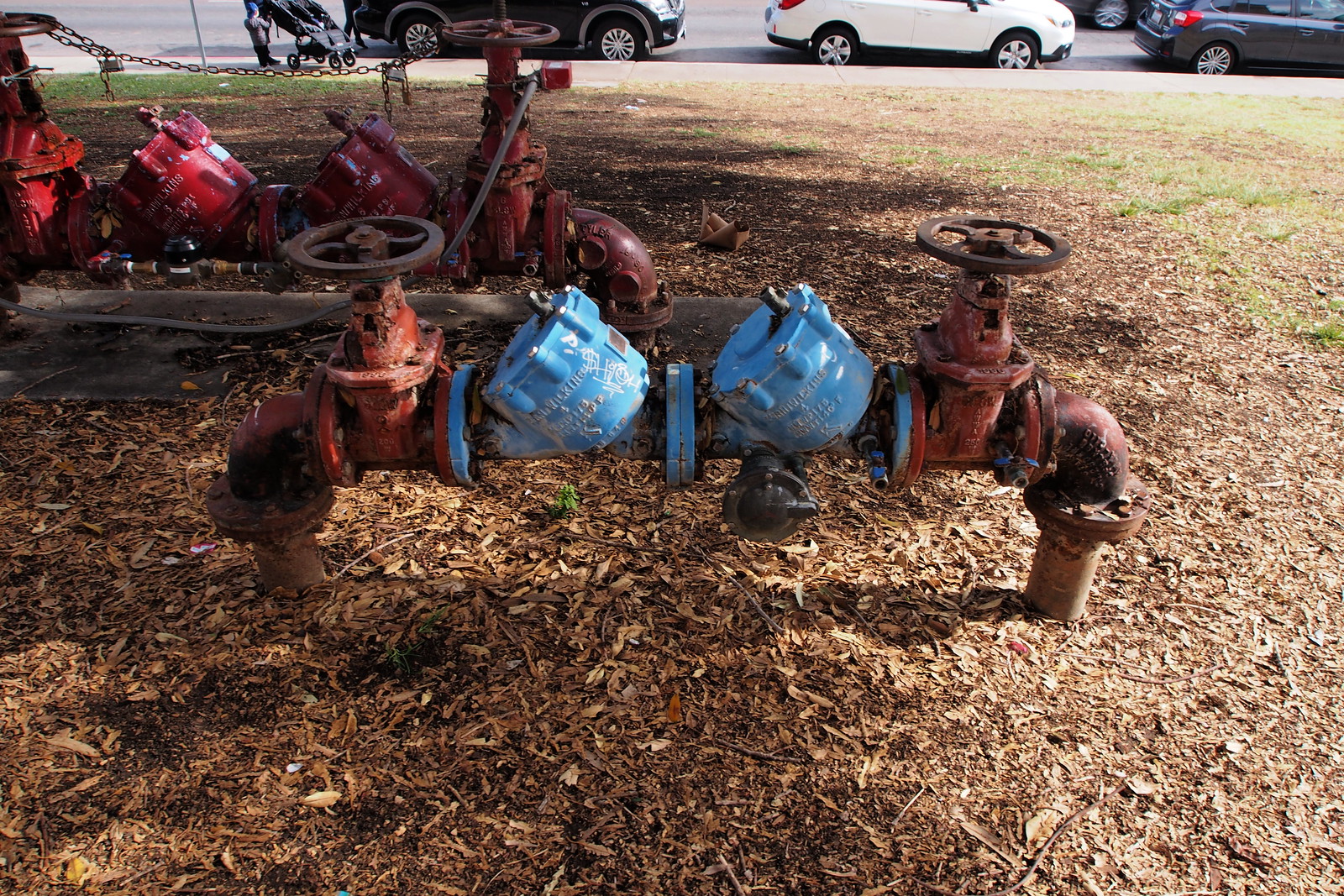The image depicts a complex drain-pipe-related machinery setup with prominent red piping and wheel valves. Emerging from the ground, the primary set consists of left and right brownish-red pipes, each capped with a red steering wheel valve. Between the valves are two blue, bucket-like structures that bear indecipherable text and have graffiti tagging on the left one. In the background, there's a nearly identical apparatus featuring red cylindrical components instead of blue ones, situated on a concrete sidewalk. The ground around the foreground machinery is marked by dry leaves and patchy grass, contrasting with the surrounding urban elements. Multiple cars—specifically black, white, and navy blue—are parked on a gray asphalt road behind the pipes, along with another grayish vehicle. Additionally, a person appears to be pushing an empty double stroller on the sidewalk, near a child standing to its left.